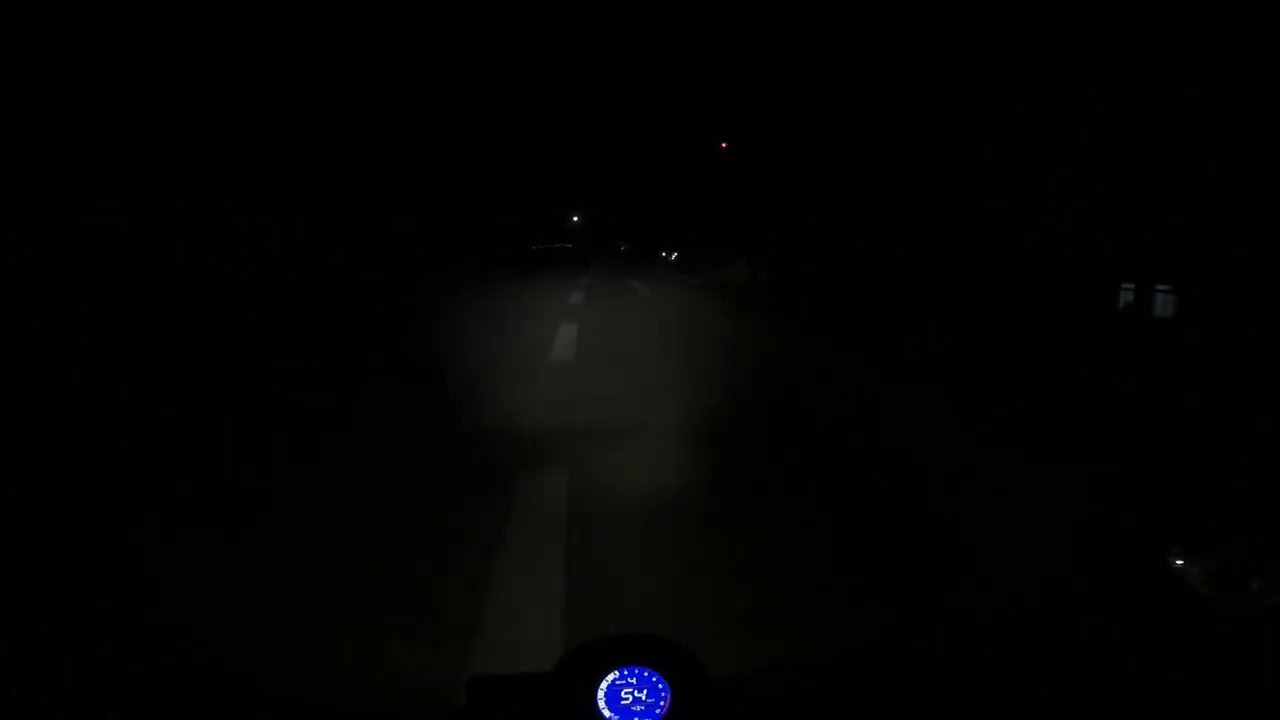The image is a nighttime scene from the point of view of a motorcyclist driving on a dark, pitch-black road. Apart from the singular illumination from the motorcycle's headlight, everything is enveloped in darkness, obscuring any details beyond the immediate foreground. The bottom center of the image features the motorcycle's electronic speedometer, displaying a white number "54" on a softly-lit blue circle. The faint outline of the motorcycle's handlebars can be just made out at the bottom of the image. Dominating the center and extending forward are the white dashed lines of the road, visibly guiding the rider down the lane. In the distance, three white lights are visible ahead, along with a single red light in the sky. The sides of the image remain pitch black, with a faint glow emanating from the lower right corner, suggesting some undefined light source. Overall, this nighttime ride is shrouded in darkness, illuminated sparingly by the headlight and the subtle electronic glow of the speedometer.